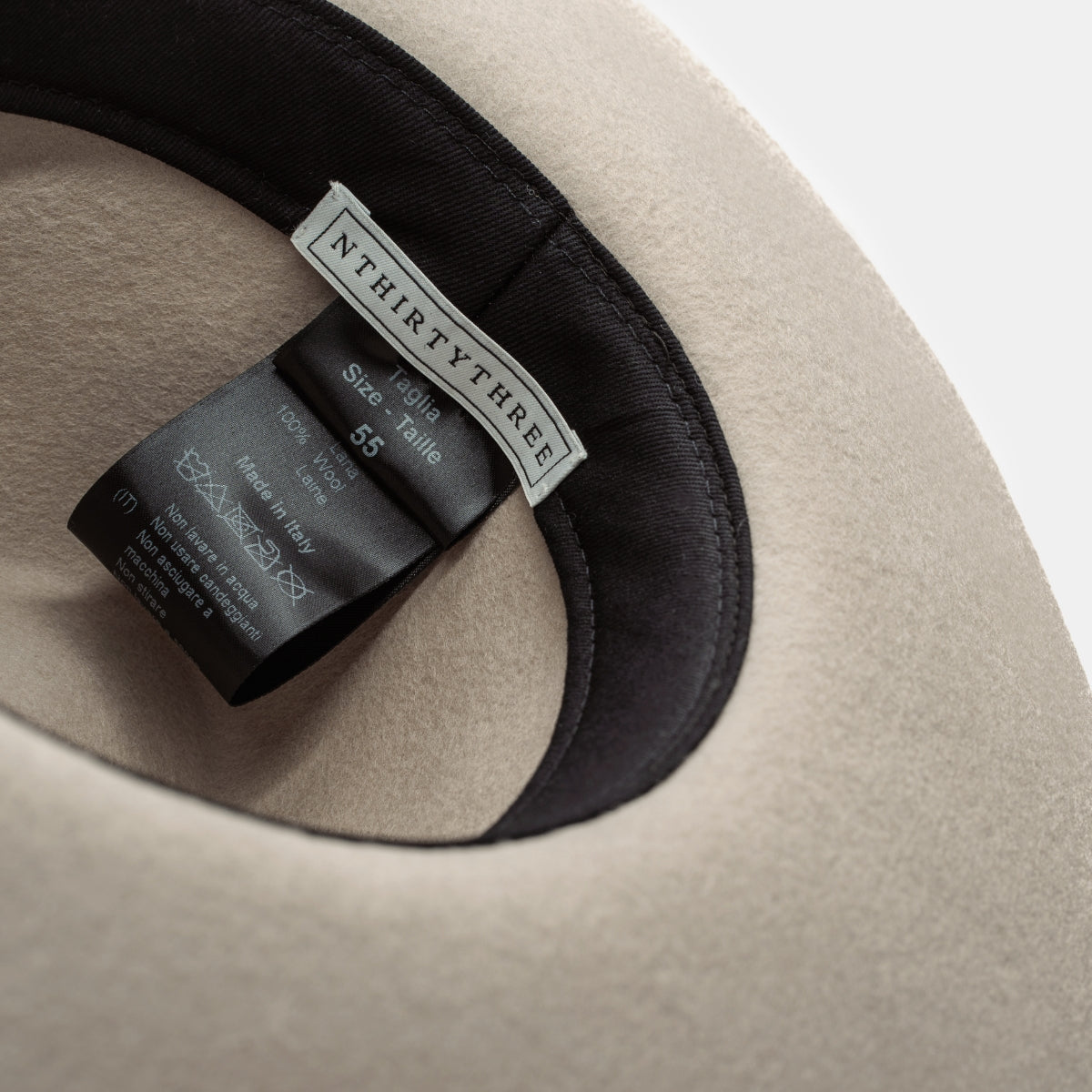This is a detailed photograph of the inside of a brimmed hat, focused on the tags and features within. The hat, which appears to be akin to a cowboy hat, is crafted from felt and is a cream or very light brown in color, almost like a pearl. It is positioned upside down, showcasing the underside where the head fits. You can see a bit of the brim encircling the hat's interior, which is lined with a dark brown or black fabric band. 

A prominent tag made from white cloth is pinned onto this band, displaying the text "N33" in capital letters. Below this tag, a black sateen tag reads "Taglia Size 55." Additionally, there is another tag providing care instructions, indicating the hat is made of 100% wool with "lain" and "lana" written on it and specifying that it is made in Italy. The instructions on this tag are printed in Italian. The entire inner lining is smooth, soft, and light brown, much like the exterior. The various labels and the felt texture underscore the hat's craftsmanship and origin.